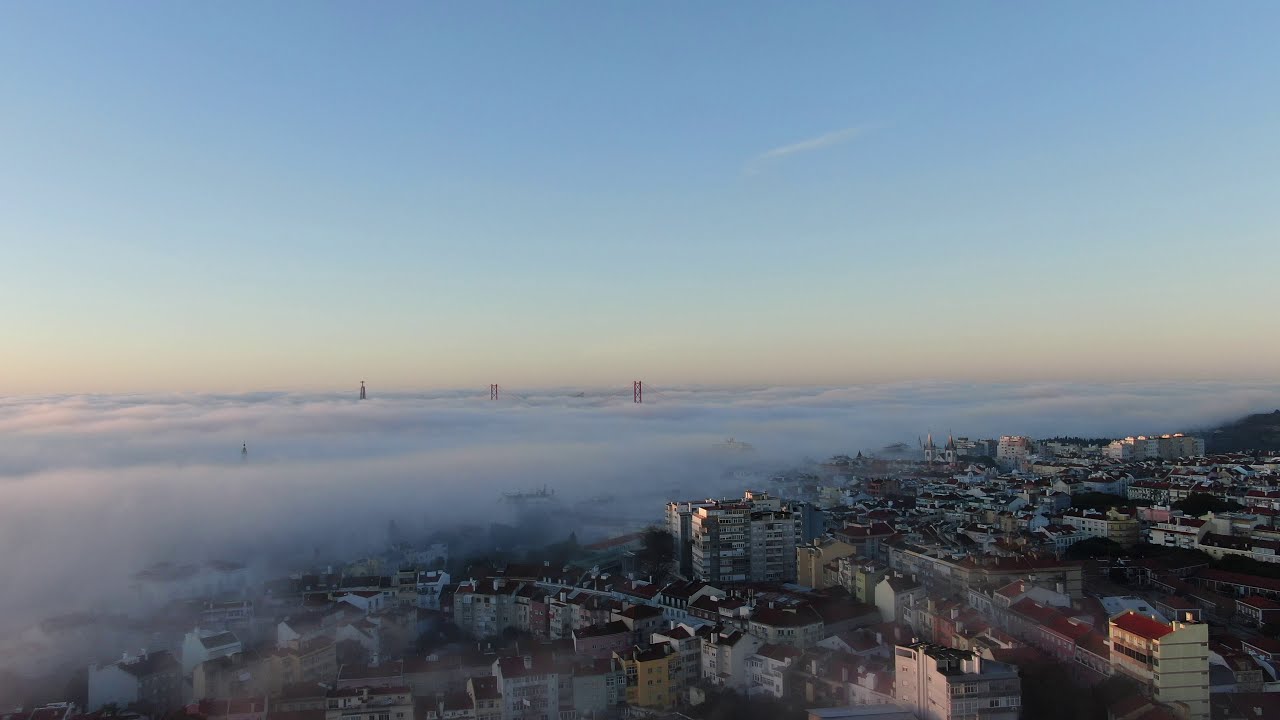This aerial photograph captures a sprawling cityscape enveloped in a foggy haze under a gradient sky transitioning from blue to pink hues. The scene reveals a densely packed urban area dominated by various multi-story buildings, ranging from six or seven stories to towering structures with dozens of floors, some topped with red roofs. The chimneys punctuate the flat roofs, enhancing the bustling appearance of the city. In the bottom right corner, the buildings stand clearly, while towards the left, they gradually succumb to the encroaching fog. Amidst this fog, the iconic three towers of the Golden Gate Bridge emerge prominently, standing in stark contrast to the shrouded city below. The far background showcases hints of mountainous terrain and the constant play of city buildings stretching into the horizon, giving a sense of depth and scale to the scene.